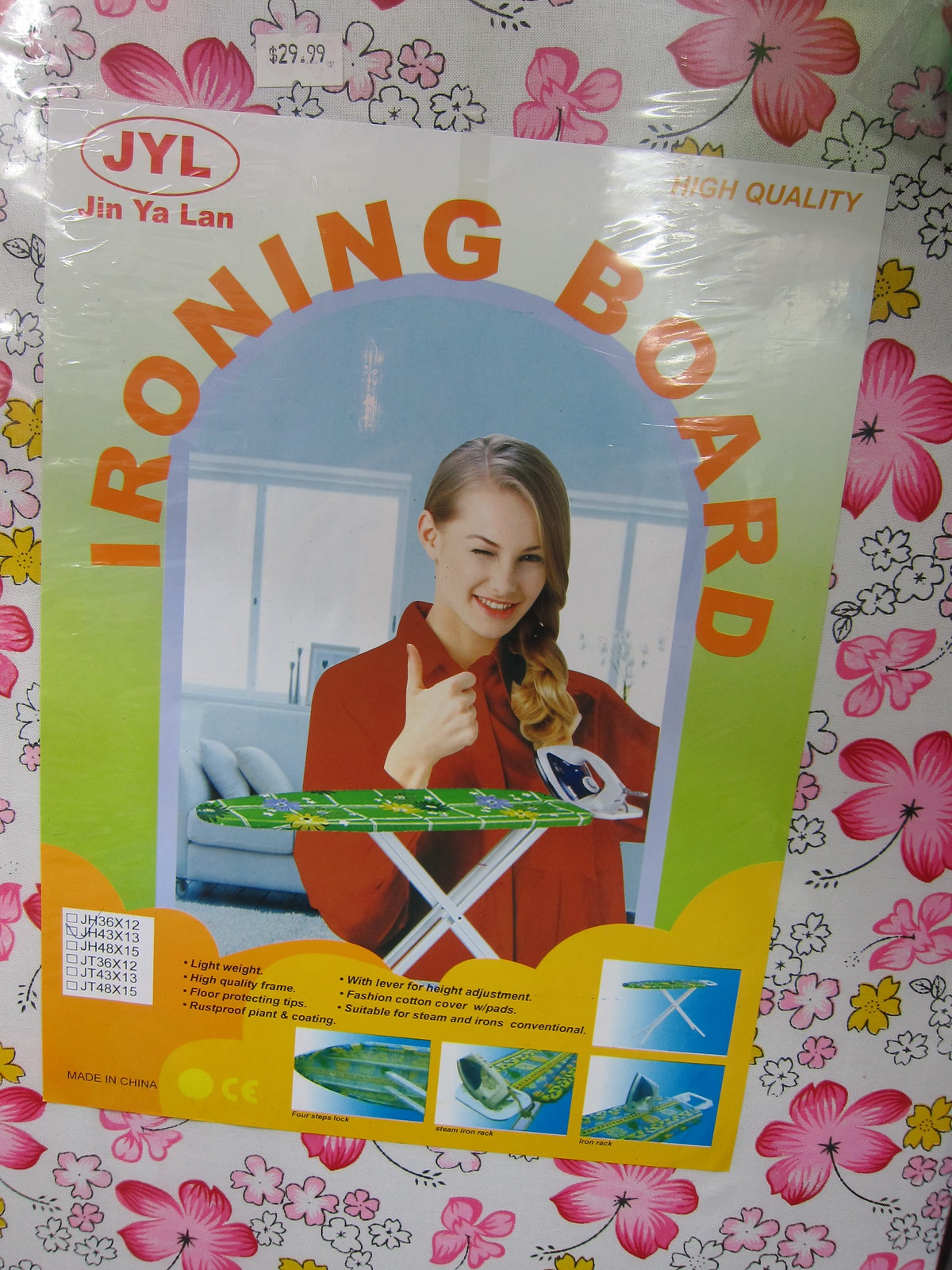The image shows a close-up advertisement for a small ironing board, sealed in clear cellophane packaging. The central focus is a photo of a smiling woman with long, blonde hair in a red long-sleeved shirt, giving a thumbs up with her left hand. She stands behind the ironing board, which is covered in a floral-patterned fabric. The cover's design features dark green fabric with dark blue, purple, yellow, hot pink, and white flowers. 

Above the woman's picture, bold orange text reads "IRONING BOARD" in an arc, while a red circle to the side contains the initials "J-Y-L," and the name "Jin Ya Lan" appears just below it. Additionally, the phrase "HIGH QUALITY" is in the upper right corner. The bottom section of the image includes model numbers and a legend listing features: "Lightweight," "High Quality Frame," "Floor Protecting Tips," "Rust Proof Paint Coating," "Width Lever and Height Adjustment," "Fashioning Cotton Cover with Pads," and "Suitable for Steam and Iron Conventional."

Several smaller images show the ironing board in different states: folded, standing, in use, and paired with an iron. The scene is set against a cream-colored floor, with light gray furniture visible in the background, and a price tag of $29.99 is partially visible at the edge.